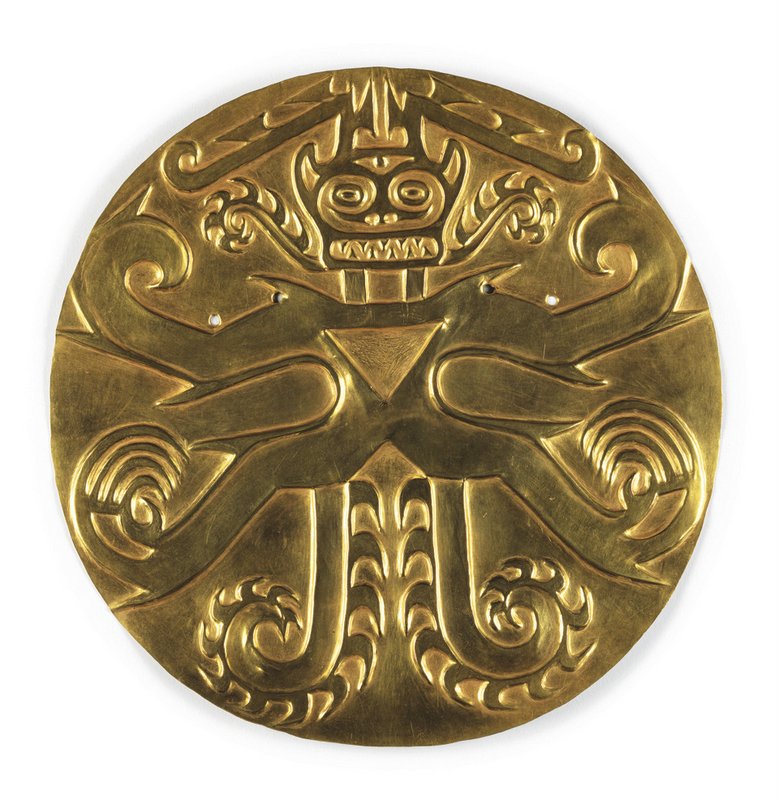The image showcases an intricately carved, large, round gold medallion, featuring a central figure with a bat-like head adorned with a crown. This figure has prominent eyes and two small, noticeable teeth at the front. The arms are spread out, ending in rounded tips, and exhibit a striped pattern of gold and black. The figure's body is highlighted by a flat, gold triangle at its center. Below this, the figure has two additional arms, each with internal spirals, and two legs extending downwards, curling upwards at the ends. The legs are adorned with small spikes along their curled sections. The entire figure, rendered in rich gold, gives the impression of a majestic and elaborate mythical creature.